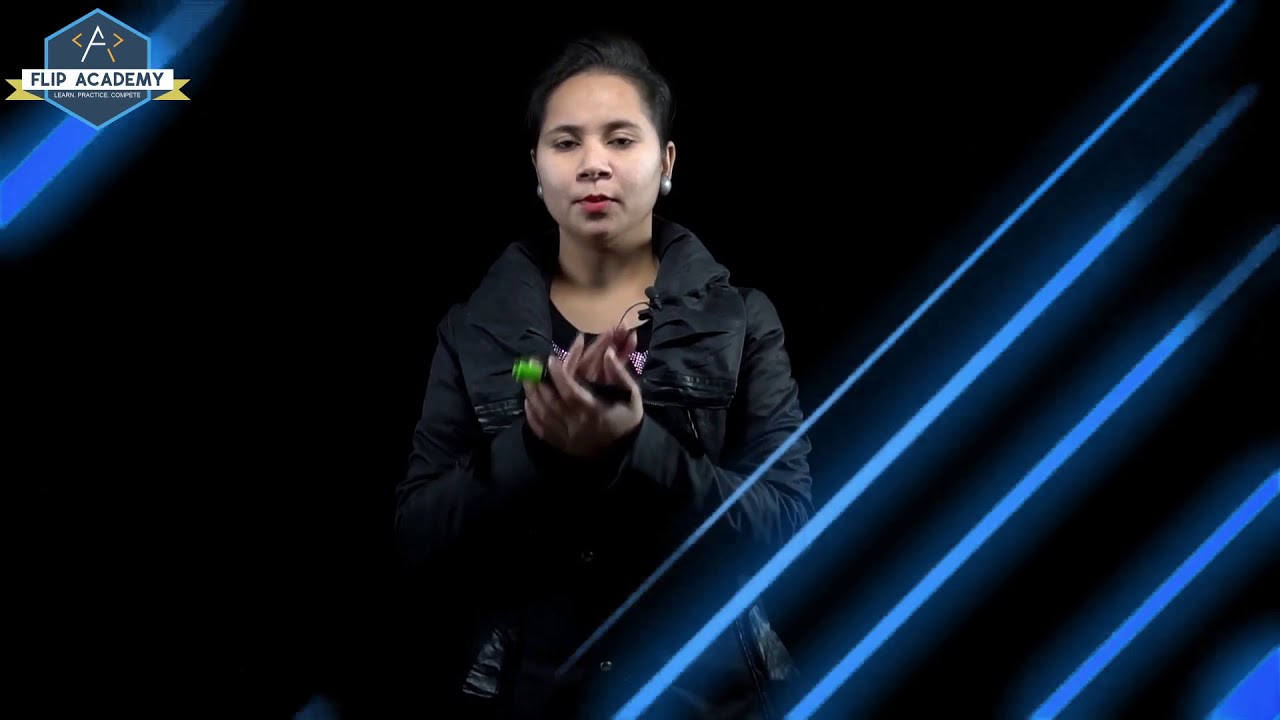The image is a detailed photograph featuring an Asian woman with dark hair that is pulled back or short, wearing pearl stud earrings. She is dressed in a heavy, dark-colored jacket, possibly black, which has a collar. In the center of the photograph, she stands with her hands in a clapped position, one hand holding what appears to be a marker with a blue or green tip. Additionally, she has a microphone clipped to her lapel.

The background is predominantly black, creating a stark contrast with the figure. There are several neon blue stripes or streaks across the background, primarily concentrated in the upper left corner and running midway through the right side of the image. In the top left corner, there is a hexagonal icon featuring the letter "A" flanked by carat symbols (<A>), with the text "Flip Academy" beneath it. Below this, there is smaller, hard-to-read text that potentially says "Levin Practice Group" along with a yellow banner. The overall setting appears to be indoors, where the woman is the focal point amidst the vividly graphic elements and dark backdrop.